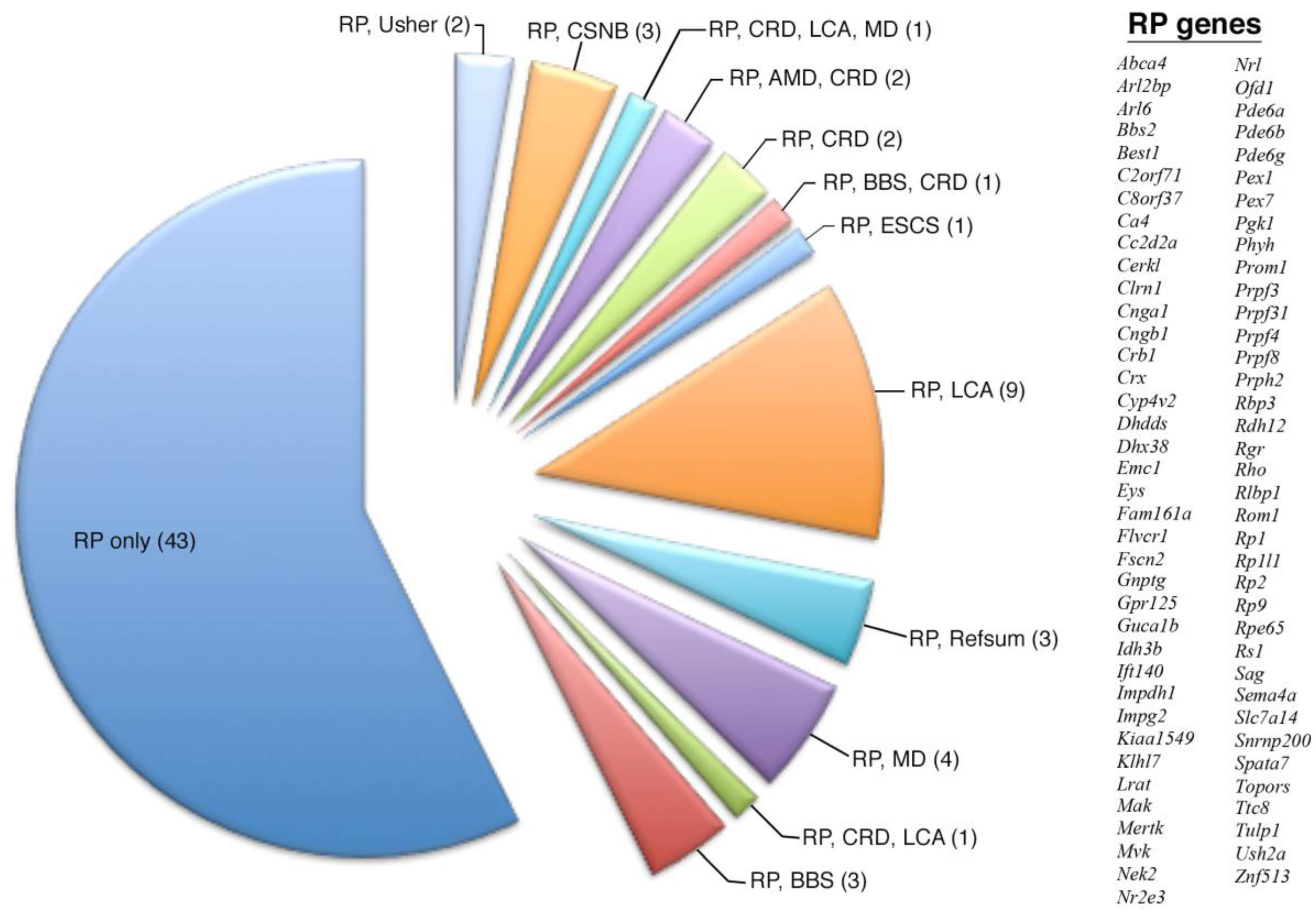This image displays a detailed breakdown of RP (Retinitis Pigmentosa) genes, likely intended for an advanced biology presentation. Centered prominently is a pie chart that visually segments various types of RP genes. The left half of the pie chart, which is the largest segment occupying approximately 55-60%, is labeled "RP only (43)" in light blue. The right half of the pie chart is divided into smaller, multicolored segments, each annotated with specific RP subtypes and their frequencies. These subtypes include names like "RP Usher (2)", "RP CSNB (3)", "RP LCA (9)", "RP MD (4)", among others, coded in colors such as light blue, light purple, light green, and light pink.

Adjacent to the pie chart, on the right side of the image, is a comprehensive list titled "RP genes". This list includes over 20 different gene abbreviations, all italicized and arranged in two columns. Examples of these gene names are NRL, ABCA4, ARL6, and RS1, presumably contributing to the various RP subtypes depicted in the pie chart. The combination of the pie chart and the detailed gene list suggests a complex analysis of genetic involvement in Retinitis Pigmentosa, indicative of a high-level biological or biochemical study.